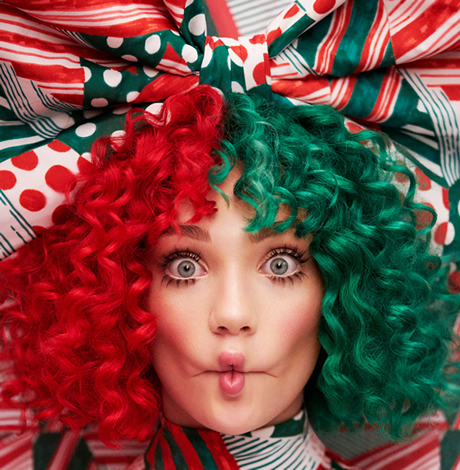This detailed color photograph captures a close-up headshot of a white woman with curly, chin-length hair that's divided into vibrant halves—red on the left and green on the right, both adorned with bangs. Her striking blue eyes and long eyelashes are accentuated as she purses her lips in a playful fish-mouth expression. She is either wearing or surrounded by an elaborate, multi-patterned fabric that matches her eccentric hairstyle. The fabric features a mix of red and white stripes, green and white stripes, and green sections with large white dots, creating a festive, patchwork-like backdrop. It appears to be wrapped around her neck and possibly forms a large, colorful bow above her head, integrating seamlessly with her vivid appearance. The coordinated fabric design extends to her collar, ensuring that the red and green theme is consistently maintained throughout the photograph.